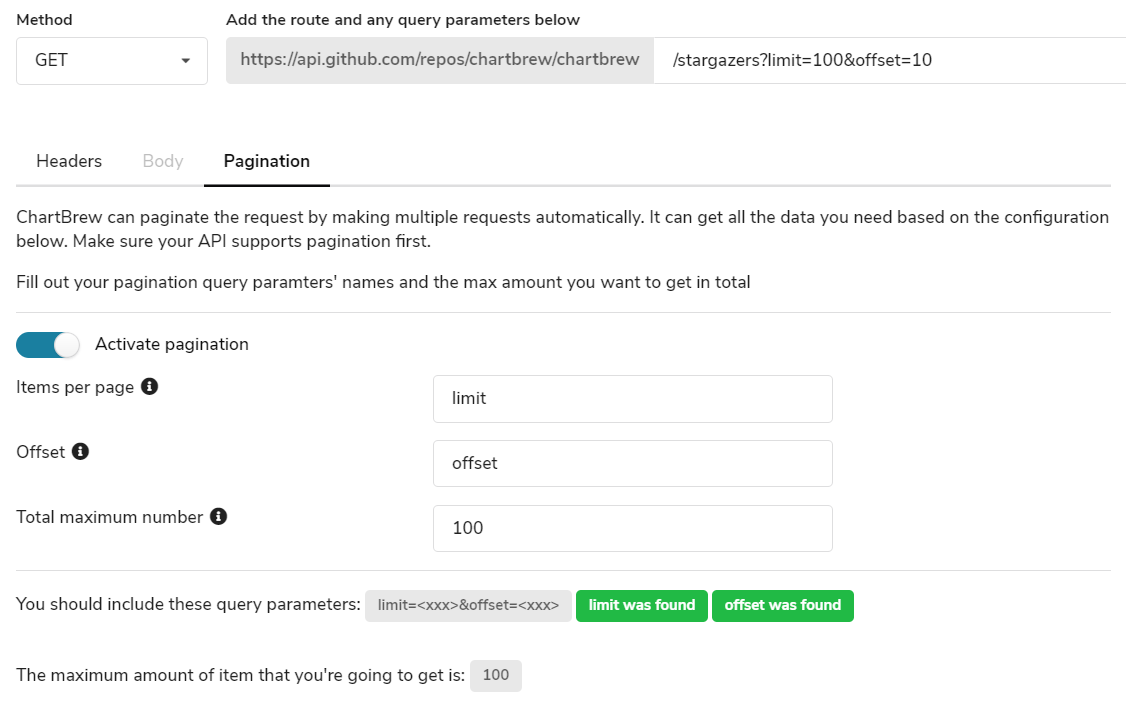This image is a screenshot from GitHub, showcasing the use of the program ChartBrew. At the top left, there is the "Method" option set to "GET". Below that, there is an instruction that reads "Add the root and any query parameters below", followed by a URL: "https://api.github.com/repos/ChartBrew/ChartBrew". This URL is extended in a white input box to include "/stargazers?limit=100&offset=10".

Beneath this section, three headings are visible: "Headers", "Body", and "Pagination". The text under "Pagination" states: "ChartBrew can paginate the request by making multiple requests automatically. It can get all of the data you need based on the configuration below. Make sure your API supports pagination first."

There is a detailed guide on filling out pagination query parameters, including their names and the maximum amount of data to retrieve. The "Activate Pagination" button is engaged. For "Items per page," the term "limit" is indicated, while for "Offset," the term "offset" is shown. The total maximum number is set to 100. At the bottom right of the image, two buttons confirm that "Limit was found" and "Offset was found."

This detailed interface allows users to efficiently manage API requests and data retrieval using ChartBrew's pagination features.